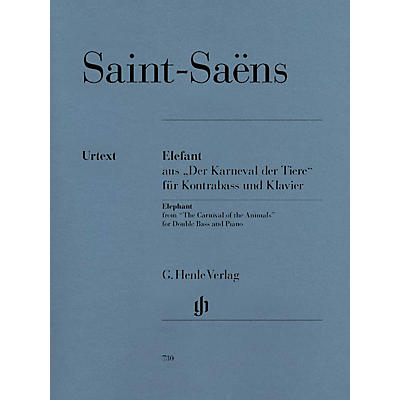The image is a cover of a music book with a grayish-blue background and plain black lettering, devoid of any designer graphics. At the top, in the largest font, it reads "Saint-Saëns," with the letter 'e' bearing two dots above it. Below this, there are three lines of text separated by black lines. The second line, in slightly smaller font, includes both German and English texts: "Urtext Elefant aus der Karneval der Tiere für Kontrabass und Klavier," translating to "Elephant, from The Carnival of the Animals, for double bass and piano." Below this, the third line features the author's name, "G. Henle Verlag," followed by a symbol or logo consisting of the initials "G" and "H." The text is all in Times New Roman font, and at the very bottom, there is a small, unreadable number "710."